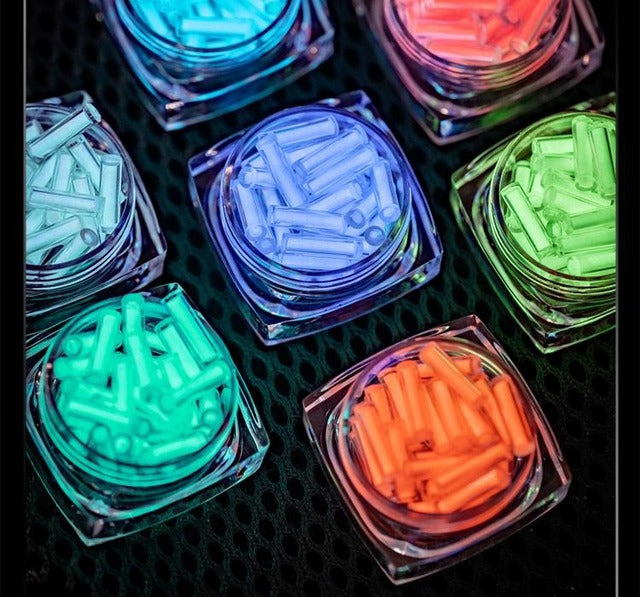The image features seven glass containers, each filled with various colored glass beads, arrayed in a circular formation with six surrounding one central container. The neon blacklight-sensitive beads range in color from neon green, teal, purple, neon aqua, neon red, orange, to multiple shades of blue, including light blue and a lighter sky blue. These tube-like beads, similar to elongated perler beads, glow vividly under the blacklight, enhancing their vibrant colors. The containers themselves resemble small, empty blush containers, square in shape with circular openings. They are set against a dark, grating-patterned background, which subtly highlights the high-contrast, glowing colors of the beads.